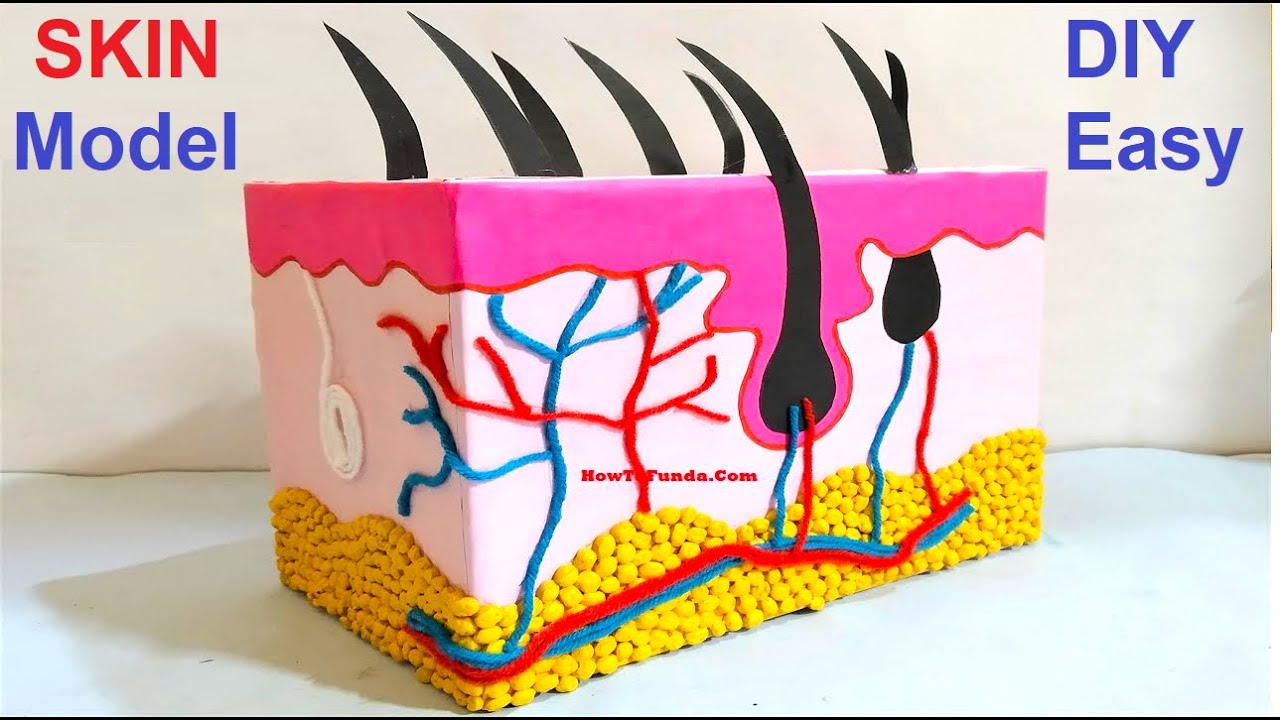In this horizontally-oriented rectangular image, we see a digitally created diagram set against a white background. In the upper left corner, the word "skin" is displayed in red print while "model" is in blue print. The upper right corner features the phrase "DIY easy" in blue print. Central to the image is a three-dimensional, cube-like representation of the skin's layers, resembling a meticulously crafted clay model. The topmost layer is depicted in pink, transitioning down to a white middle layer, and culminating at the bottom with a yellow layer composed of elements that resemble tiny corn kernels, representing the subcutaneous fat. Printed discreetly in red text at the center of the skin model is the website "howtofunda.com." Emerging from the pink layer of the skin model are a few spiky black hairs, which are bent and angled diagonally to the left.